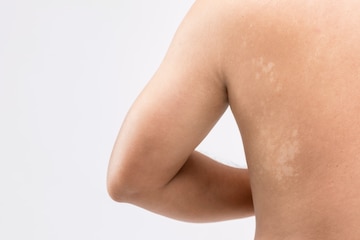This horizontally-aligned, zoomed-in photograph captures the left-side profile of a white-skinned person with a slightly tanned complexion. The image, featuring no visible body hair, focuses on the person's back and arm, set against a light gray, featureless background. The shot extends from just below the top of the shoulder to partway down the ribcage, clearly displaying the shoulder blade, elbow, forearm, and the upper arm forming a triangular space against the body. Noticeably, the skin on the back reveals several splotchy sections with varying pigmentation, possibly indicative of scar tissue or old rash marks. The primary emphasis is on these skin discolorations, suggesting a medical context such as a dermatological examination. The photograph is devoid of text and other subjects, keeping the focus entirely on the individual's back and the details of their skin condition.